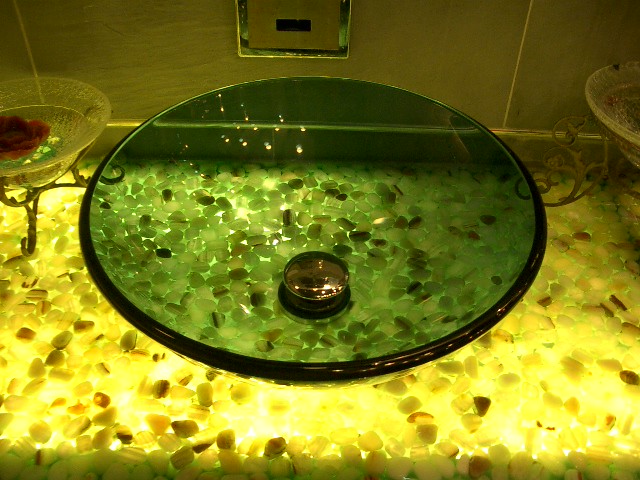In this colorful landscape photograph, the foreground is dominated by an array of small, smooth, irregularly shaped stones, bathed in a bright yellow glow emanating from beneath them. Resting on these stones is a small, round base supporting a large green glass bowl with a dark rim. The clarity of the green glass allows a view of the yellow stones underneath, which take on a greenish hue through the tinted bowl. In the left corner of the photograph, there is a clear glass bowl with ornate iron legs that intricately curl upwards at the edges. At the center of this bowl, a vibrant red, rose-like flower adds a contrasting splash of color. On the right side of the image, another clear glass bowl with similarly ornate legs is visible, though it is cropped in such a way that the contents remain hidden, adding a sense of mystery to the scene.